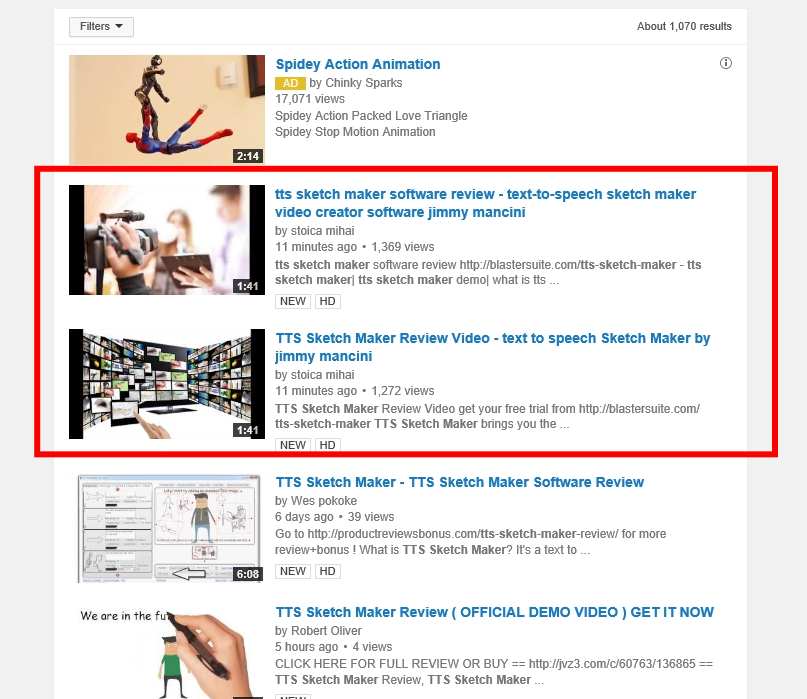This is a detailed screenshot displaying various options available in the SketchMaker software interface. At the very top, an advertisement for "Spidey Action Animation" features what appear to be two bendable action figures in a dynamic pose, suggesting they are in the midst of a fight. Below the advertisement, the first thumbnail image shows a person holding a camera, another person holding a script, and a third person who is faintly visible in the blurry background. The following thumbnail preview illustrates what appears to be a library or gallery of images. Next in line is an image of a cartoon man, likely indicative of a section dedicated to creating different character designs. The subsequent thumbnail showcases a hand writing the phrase "We are the future" with a pen, accompanied by a cartoon character wearing a green shirt positioned below the text. These thumbnails are aligned vertically down the left-hand side of the interface. Centered in the image are detailed descriptions of various choices for videos and resources related to SketchMaker's text-to-speech features and other functionalities of the software.